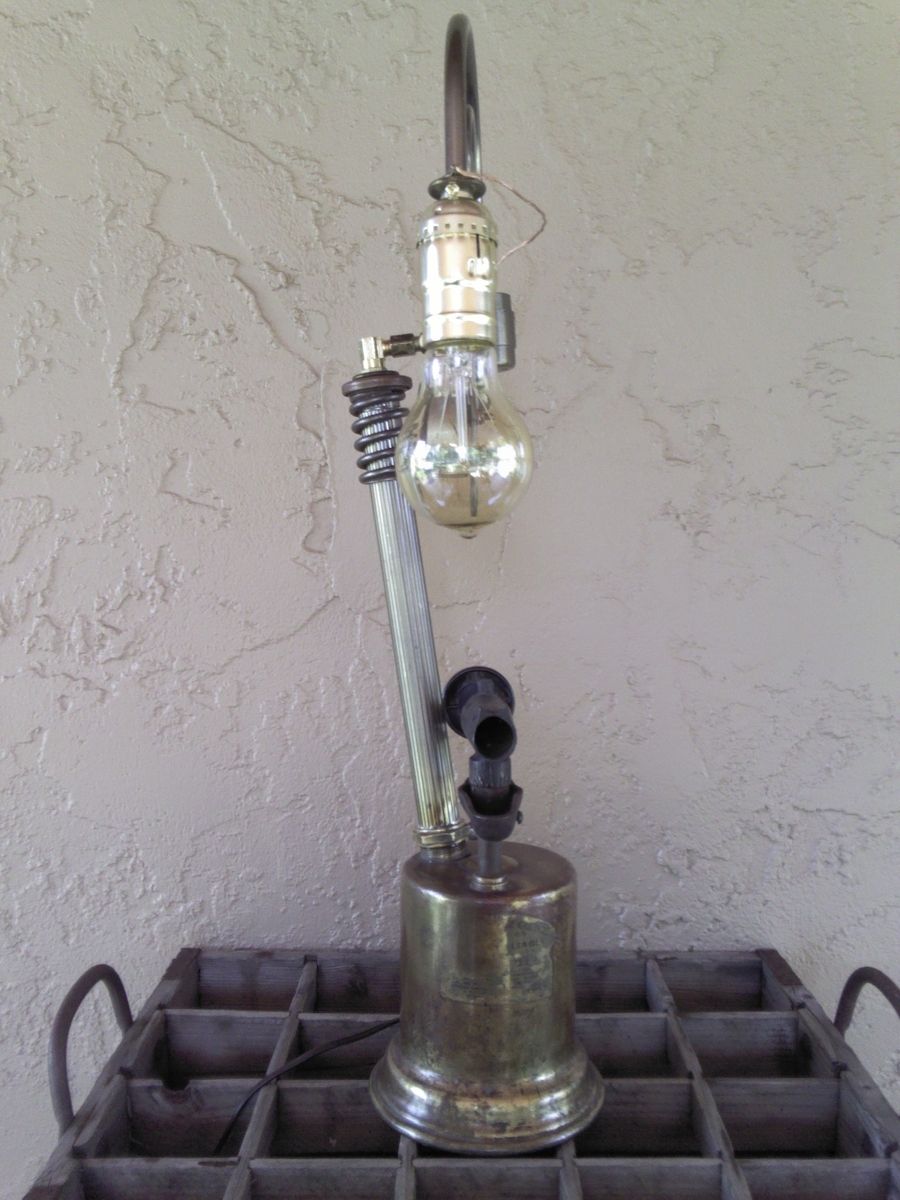Close-up image of a homemade table lamp device set on top of a cart with a square grid surface. The background is a poorly painted, cracked, and peeling white stucco wall. The lamp consists of a metal can serving as the base, from which a plumbing fixture extends. This fixture is connected to a rod with a right-angled fitting that supports a second fitting, bending over to hold an exposed, downward-facing incandescent light bulb with a slight brownish tint. The lamp's components include varied items like a black attachment, a white attachment with a spring core, and other improvised parts, giving it a makeshift and experimental appearance. There is no shade on the light, and the colors of the lamp's elements include brass, silver, and gold, suggesting it is a crafted, inventive piece.